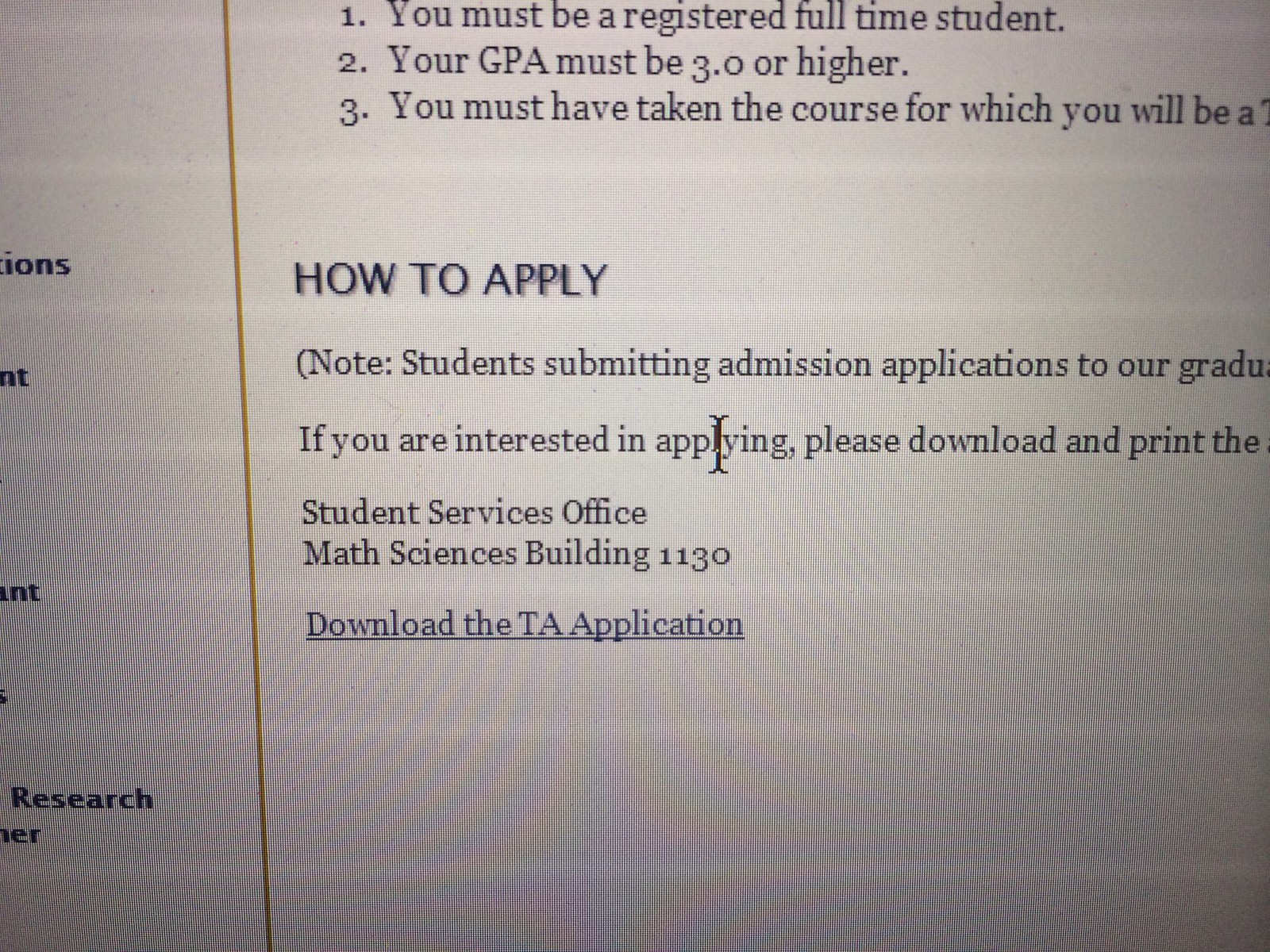The image appears to be a photograph of a computer screen displaying partially visible information on a white background. The image is grainy, suggesting it was taken with a phone or digital camera. On the left side, there is incomplete text divided by a vertical orange line. The legible information on the right side includes application requirements and instructions: "Number one, you must be a registered full-time student. Number two, your GPA must be 3.0 or higher. Number three, you must have taken the course for which you will be a," followed by the word "how to apply." The section reads further, "Note: Students submitting admission applications to our graduate," and then is cut off. Additional legible text includes, "If you are interested in applying, please download and print the," followed by "Student Service Office, Math Sciences Building, 1130," and finally, "download the TA application." A cursor is visible over the word "applying," indicating potential interaction with the text.